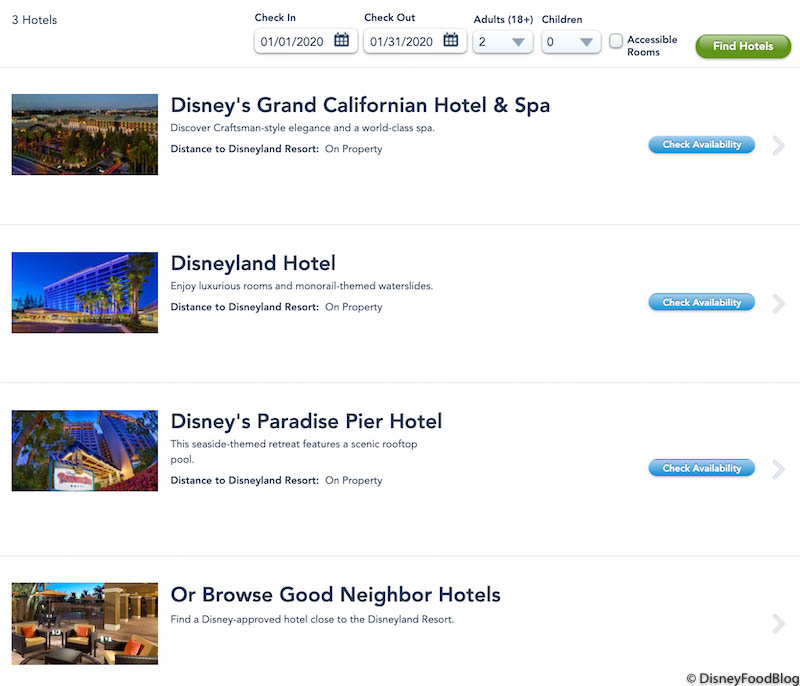This detailed caption should help:

"In this informative screenshot from a website (credited to Disney Food Blog) located in the bottom right corner, viewers can see a Disney hotel booking interface. At the top, there are fields for selecting check-in and check-out dates, along with drop-down menus for specifying the number of adults and children. An unchecked box labeled 'Accessible Rooms' is present, followed by a 'Find Hotels' button situated to the right. Below this section, the first hotel listed is Disney's Grand Californian Hotel and Spa, followed by Disneyland Hotel, Disney's Paradise Pier Hotel, and a section for Orbrow's Good Neighbor Hotels which invites users to find Disney-approved accommodations near Disneyland Resort. Each hotel listing on the right side features a 'Check Availability' button in blue, alongside photos of the hotel's exterior. The names of the hotels are presented with concise descriptions underneath the images, offering users a visual and textual overview of each option."